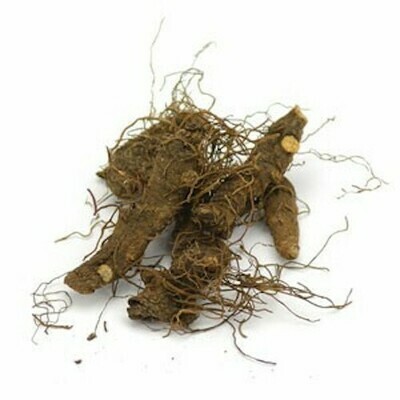The photograph displays an uncleaned, tangled cluster of substantial, irregularly shaped roots, potentially resembling tuber plants like ginger. The roots are primarily dark brown with sections of light brown, showcasing areas where they've been newly cut, exposing their lighter interior. The cluster consists of approximately 4 to 5 main roots with numerous smaller tendril-like offshoots extending in all directions, creating an intricate, web-like appearance. Notably, two of the roots have distinctive yellow knobs at their ends. Some roots lie atop others, adding to the disordered arrangement. The image, set against a plain white background, suggests a promotional context, yet contains no text, offering a stark, unadorned view of these freshly unearthed, earthy roots.